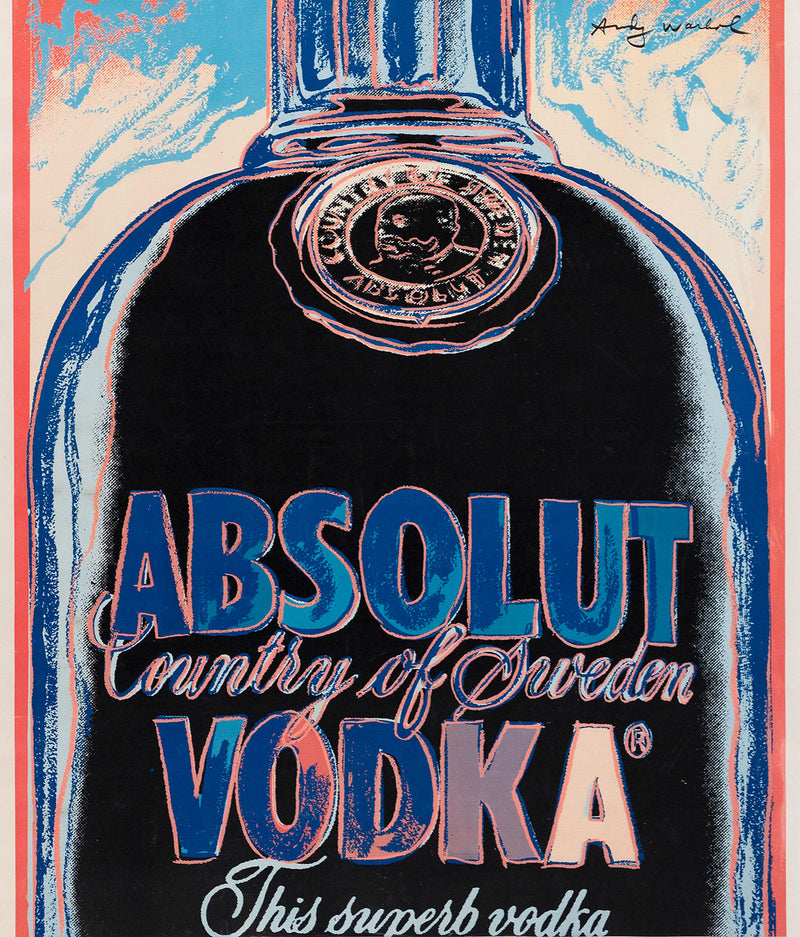This image showcases a photorealistic, pastel-like drawing of an Absolut Vodka bottle, presented in an Art Deco style. The bottle's central section is highlighted, showing off the detailed text and logo. The midsection prominently features the brand name "Absolut" in distinct blue letters, with "Country of Sweden" and "This Superb Vodka" written beneath it in a mix of blue, pink, and peach tones, outlined with various colors. The artwork reveals a meticulous attention to texture and color, with the bottle surrounded by a backdrop of swirling orange-peach, pale pink, and light blue hues. The edges of the image are bordered with grey and peach tones, enhancing the intricate design. Despite the high level of detail, the texture of the paper and the medium used indicate it is a pastel drawing rather than a digital painting, giving it a unique, almost tactile quality.